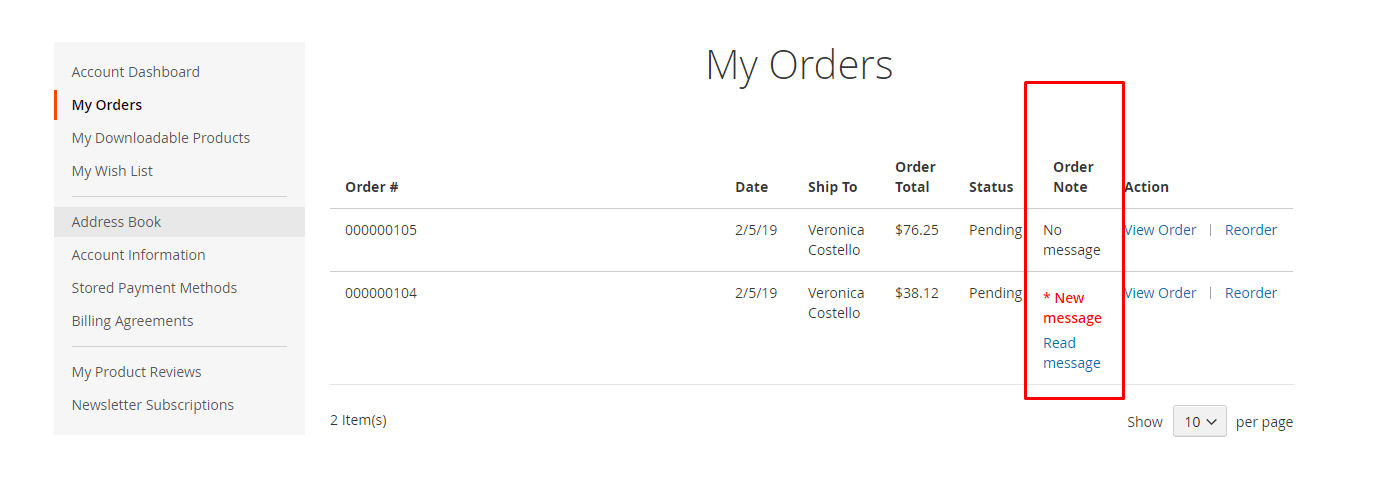**Detailed Caption:**
The image captures a screenshot of an account dashboard on an e-commerce website, showcasing a clean interface with a primarily white background. On the left-hand side, a light gray column contains a navigational menu titled "Account Dashboard," followed by various sections such as "My Orders," "My Downloadable Products," "My Wish List," "Address Book," "Account Information," "Stored Payment Methods," "Billing Agreements," "My Product Reviews," and "Newsletter Subscriptions."

To the right of this menu, the screenshot focuses on the "My Orders" section. The user has two orders listed. For each order, the details are organized into distinct columns: "Order #", "Date", "Ship To", "Order Total", "Status," "Order Notes," and "Action."

Both orders are being shipped to a person named Veronica Costello and were purchased on February 5th, 2019. The first order has a total amount of $76.25, while the second order totals $38.12. The status of both orders is marked as "Pending." Additionally, each order row provides an option to view the order details or reorder the same items.

This structured layout allows for easy navigation and clear visibility into the status and details of each order placed by the user.